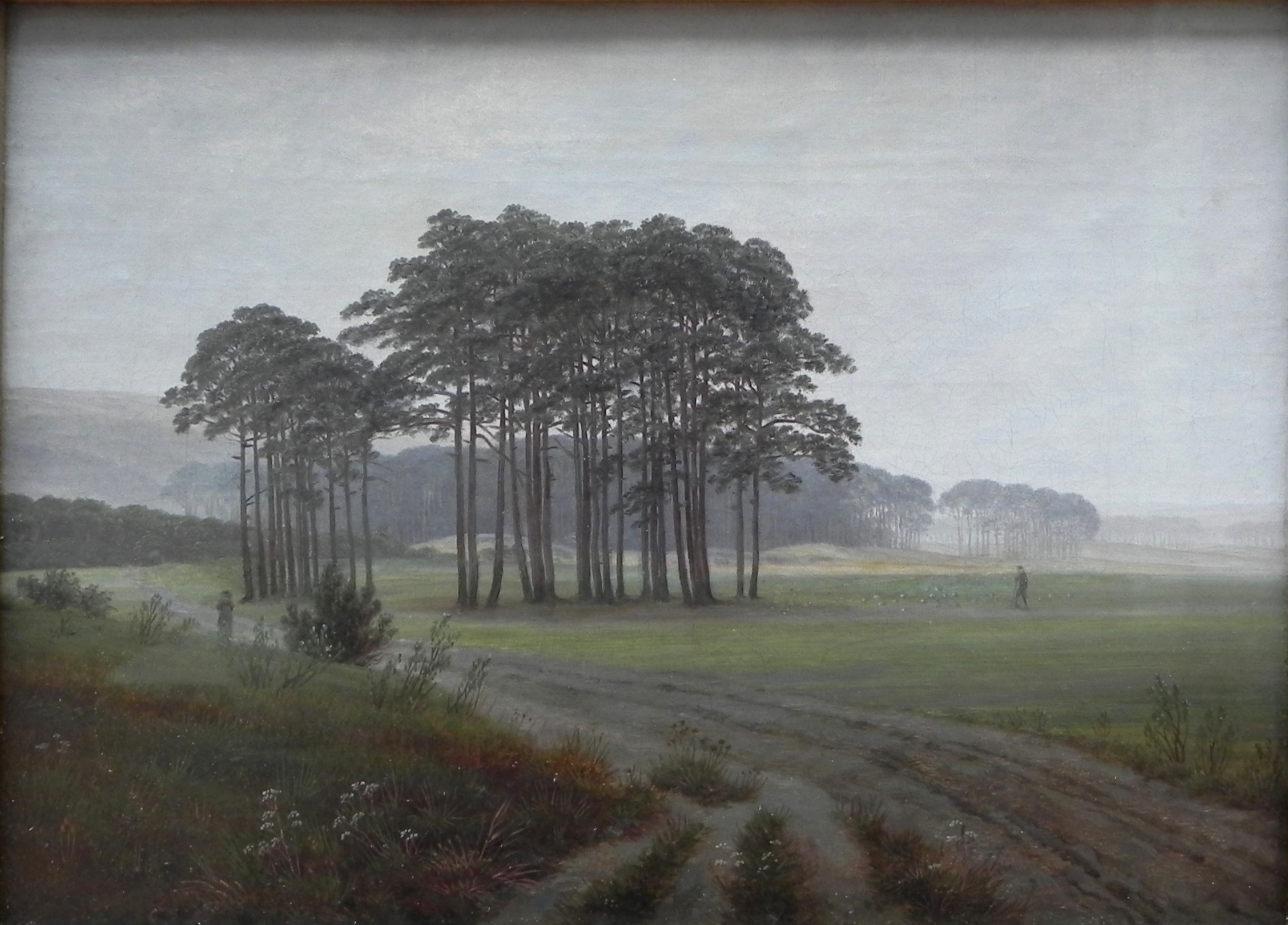The image is a detailed, likely oil-painted landscape, featuring a meandering dirt path that curves from the foreground to the left-hand middle of the scene. On the left side of the path, there's a grassy area adorned with small, white flowers. In contrast, the right side of the path showcases a wide expanse of grassland populated by multiple groups of tall, fully-leafed green trees. Two figures dressed in dark clothing appear as silhouettes: one stands far down the path toward the left, while the other is positioned to the right of the road amidst the trees. The scene is set under a light gray, somewhat blurry sky, accentuating the outdoor, serene atmosphere. In the background and flanking each side, more trees enrich the landscape, indicating a dense wooded area in the distance.